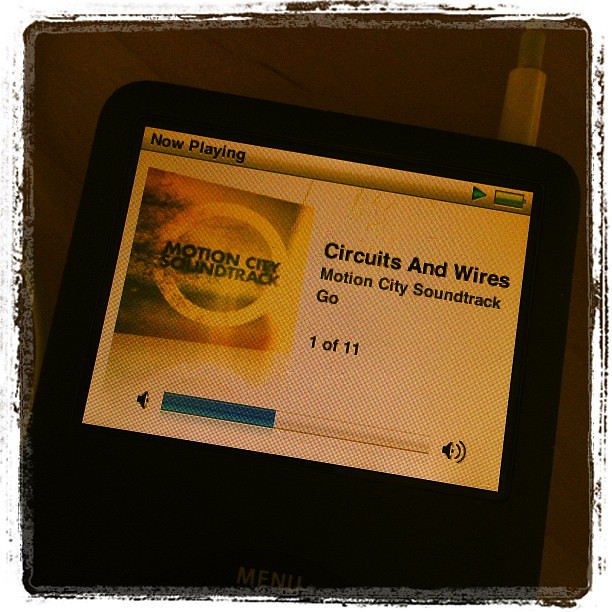The photograph is a stylized, square image dominated by a dark brown, distressed texture resembling a brush effect. At the center, an older-looking black media player, possibly an iPod or iPad, stands out against the backdrop. The player features a simplistic, rudimentary design, with a notable white headphone cord connecting at the top right. The screen displays a "Now Playing" text in black on a gray bar at the top, adjacent to a basic battery icon on the upper right. Below this, the screen shows the song "Circuits and Wires" by Motion City Soundtrack, listed as track one of eleven. To the left of the song information, there is an album cover for Motion City Soundtrack. At the bottom of the screen, there’s a volume bar set near the halfway point. The entire scene exudes a nostalgic, retro vibe, blending the tactile aesthetic of bygone technology with an early digital music experience.